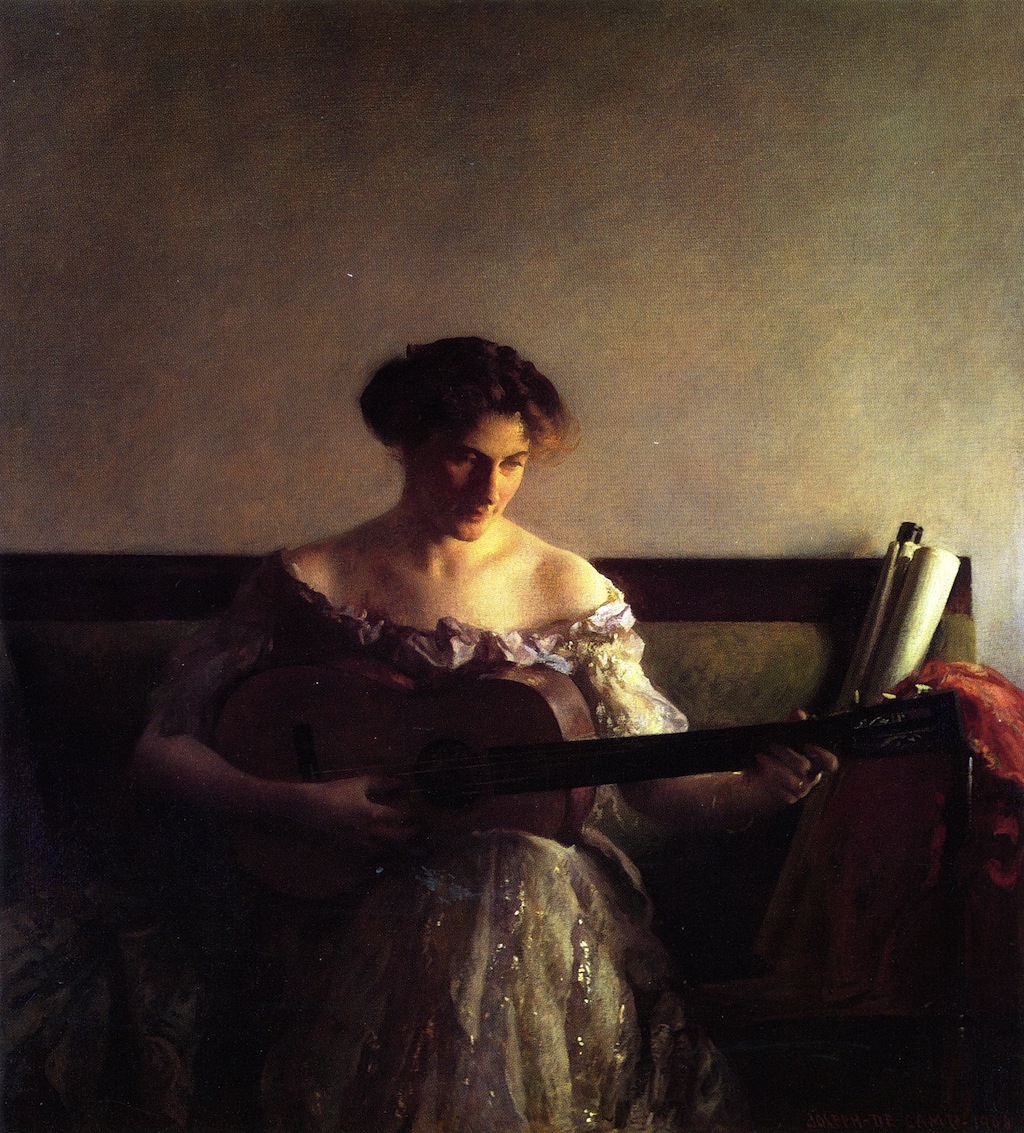In this painting, a light-skinned woman with dark hair meticulously styled around her head is depicted sitting on a green, pew-style bench with a dark brown mahogany top. The background is a nuanced blend of pale greenish and purplish tones, gradually fading into darkness at the top left corner. She is engrossed in playing a brown guitar with a dark fretboard, positioned securely on her lap. Her right arm skillfully strums the strings while her left hand expertly navigates the frets. The woman is dressed in a striking, sparkly dress that is cut low to expose her shoulders, featuring white splotches that add to its intricate design. To her right, on the bench, lies a scroll with white paper wrapped around black or brown wood, accompanied by a red blanket or garment draped over the side. The image is predominantly dark, suggesting an indoor setting and offering a somber yet intimate atmosphere.